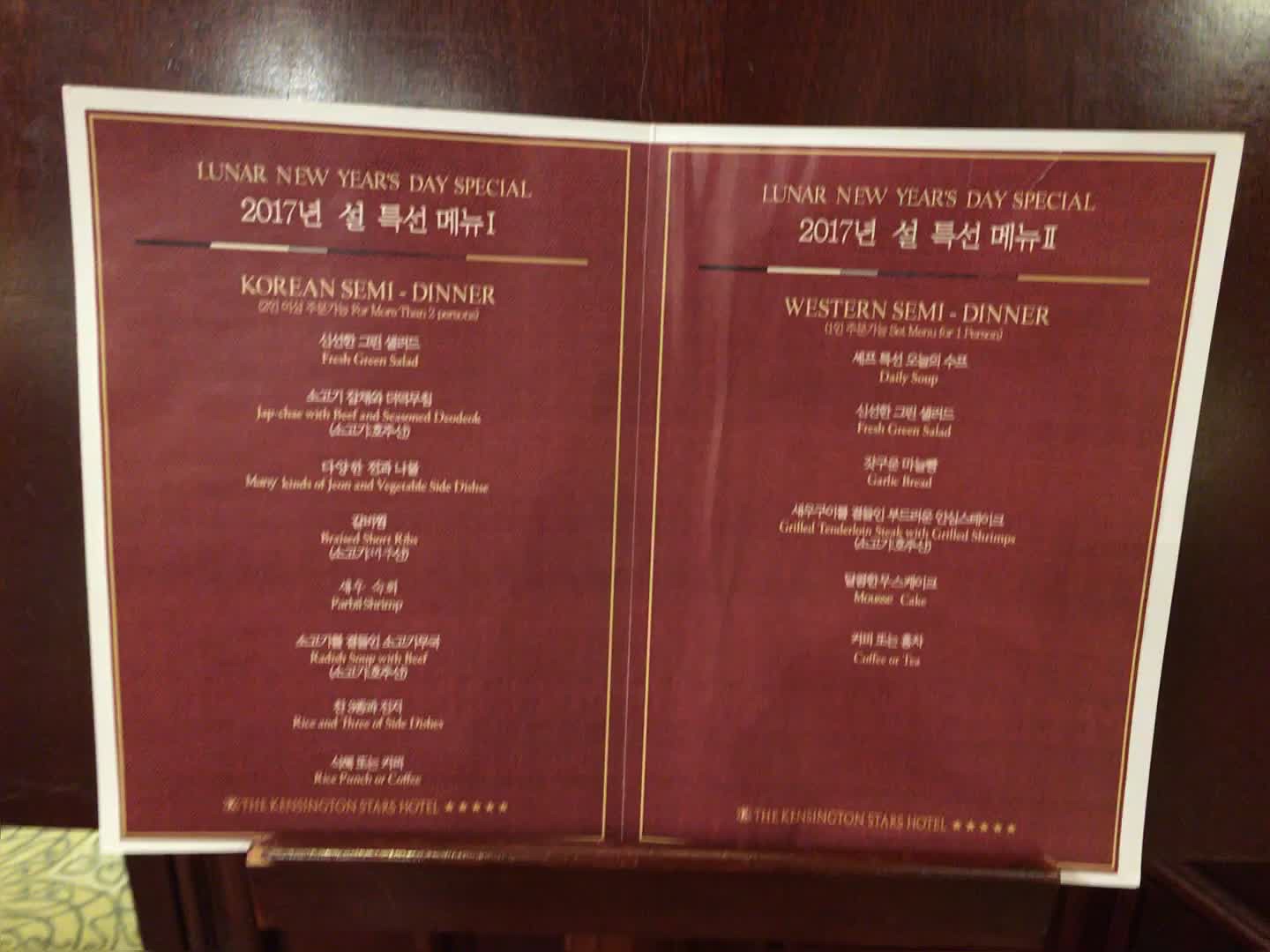The image captures a scene with a brown podium set against a background featuring light green carpet adorned with darker green swirly designs. Positioned on the podium are two side-by-side pages. Each page has a dark maroon background with a white border and pale yellow text. The left page is titled "Lunar New Year's Day Special 2017" with the subheading "Korean Semi-Dinner," followed by some illegible smaller text in an Asian script. The right page mirrors the title "Lunar New Year's Day Special 2017" but with the subheading "Western Semi-Dinner." Though the prices and additional details are not visible due to blurriness, the overall presentation suggests a special menu offering for the Lunar New Year celebration.